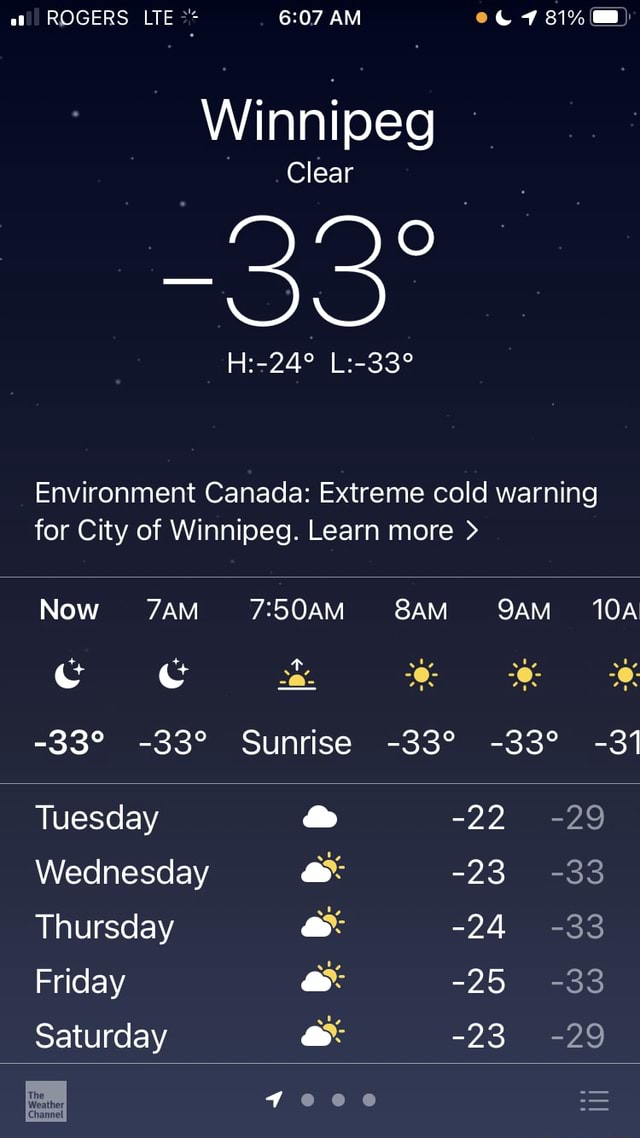The image displays a screenshot of a weather app on a cell phone screen. 

**Top Section:**
- **Top Left Corner**: Shows the connection bar, "Rogers" as the network provider, and "LTE."
- **Center**: The time is displayed as 6:07 AM.
- **Top Right Corner**: Includes a 'Do Not Disturb' icon and an 81% battery life indicator.

**Main Display Section:**
- **Background**: Predominantly black.
- **City Name**: Winnipeg, prominently displayed at the top.
- **Weather Condition**: Indicated as "Clear."
- **Temperature**: Noteworthy for its extreme cold, showing -33°C.
- **High/Low Temperatures**: High of -24°C and low of -33°C.
- **Weather Alert**: A notice from Environment Canada, marked with "Extreme Cold Warning for City of Winnipeg. Learn more" followed by an arrow.

**Hourly Forecast Section:**
- **Timeline**: From the current time up to 10 AM.
- **Temperature Consistency**: Remaining at -33°C throughout this period.
- **Weather Icons**:
  - Two moon icons for the early hours.
  - A sunrise icon in the middle.
  - Three sun icons representing 8 AM, 9 AM, and 10 AM.

**Week's Forecast Section:**
- **Daily Forecast**: Covers Tuesday through Saturday.
  - Each day starts with a cloud icon.
  - Days generally end with a mix of sun and clouds icon for the bottom row.

**Temperature Trends**:
  - **Highs**: -22°C, -23°C, -24°C, -25°C, and -23°C.
  - **Lows**: Displayed to the right of the high temperatures, though exact figures are not mentioned in the text.

**Bottom Section:**
- **Bottom Left Corner**: A square label.
- **Middle**: An arrow with three dots.
- **Bottom Right Corner**: A tab menu. 

The layout is organized to provide comprehensive weather information with emphasis on the cold temperatures and impending extreme cold warning for Winnipeg.